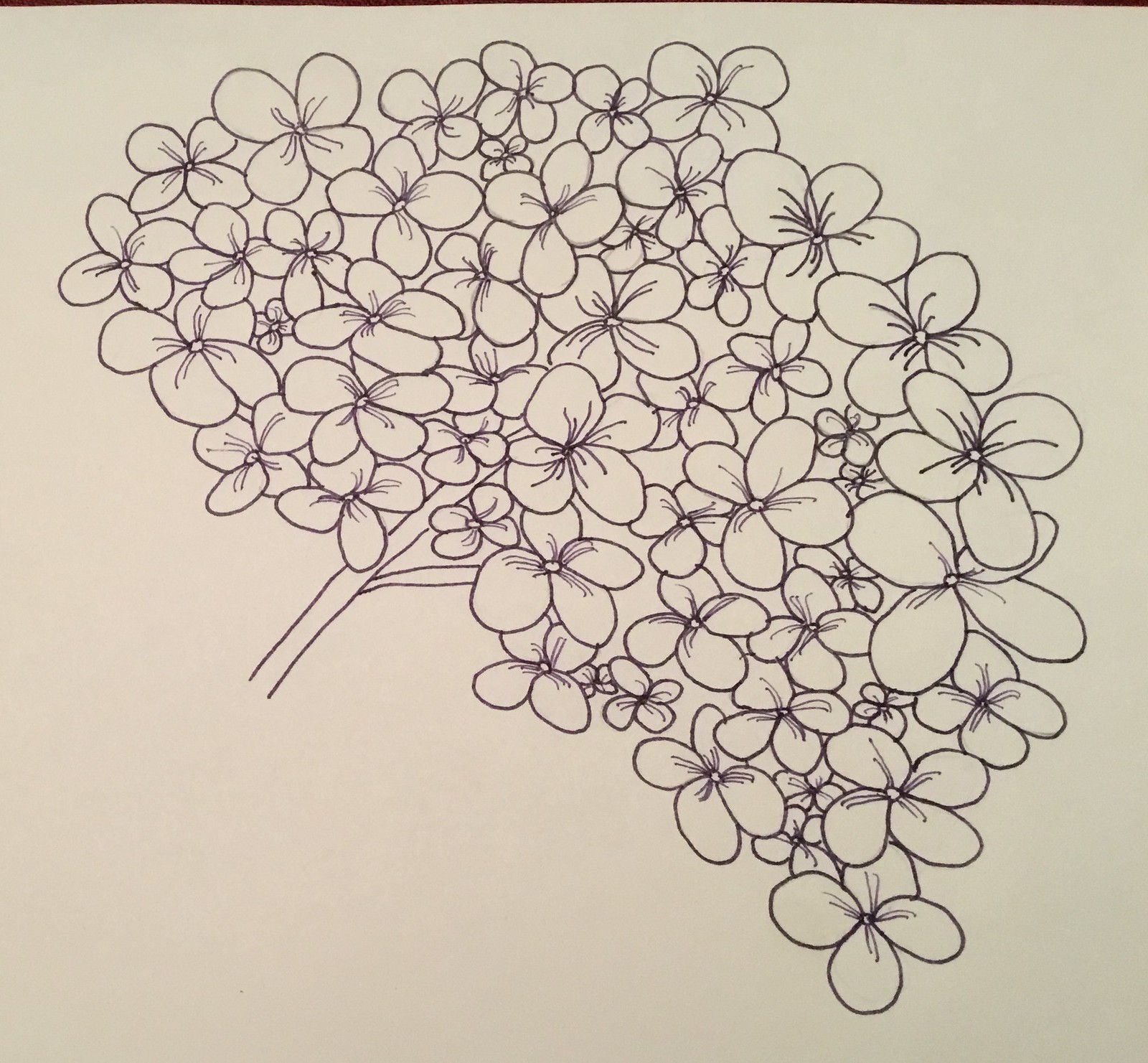This is a detailed ink drawing on a white sheet of paper, depicting the intricate structure of a flowering plant. The main feature is a branch with a smaller offshoot, adorned with dozens of clover-like flowers. Each flower is composed of four petal-like shapes, resembling four-leaf clovers, ranging widely in size from quite large to very small. The larger flowers are predominantly clustered on the left side and at the top right, while medium-sized flowers are scattered across both sides and the center mostly contains the smaller ones, although they are distributed throughout the drawing. Each petal has delicate diagonal lines emerging from a central small circle, giving them a textured appearance. Most flowers float independently in space, not visibly attached to the central branch apart from a few near the stem. The entire composition is rendered in black ink, bringing out the stark contrast between the intricate lines of the floral canopy and the clean white background.